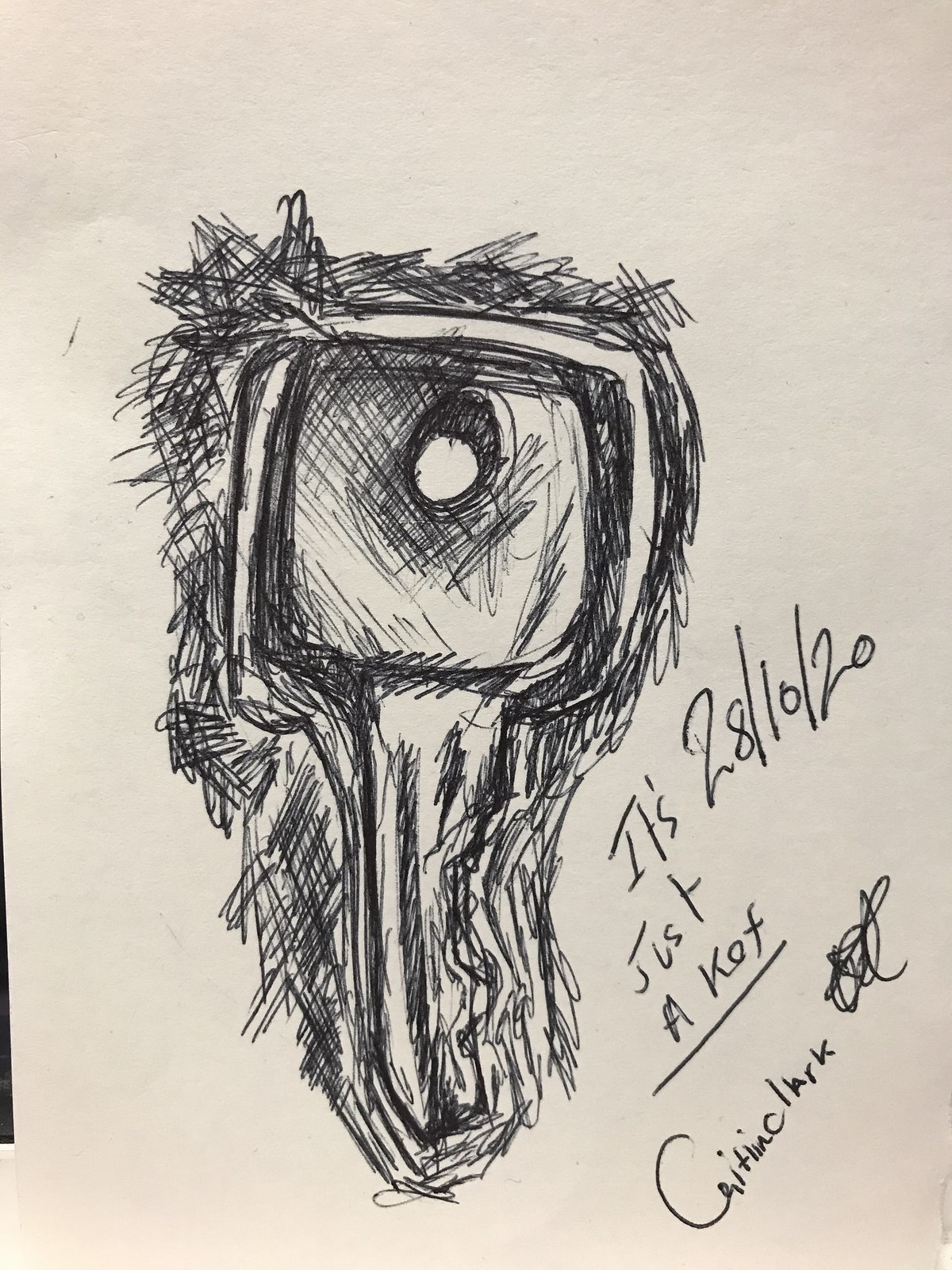The image features a white paper background with intricate black pen sketches. To the right side of the paper, the date "28/10/20" is inscribed. Below the date, the word "key" is written and underlined. The center of the image appears to be dominated by a square with a hole in the middle, representing a keyhole. At the bottom of the sketch, there is a depiction of a key. The entire scene is surrounded by various scratch marks, adding a sense of texture and complexity to the artwork.